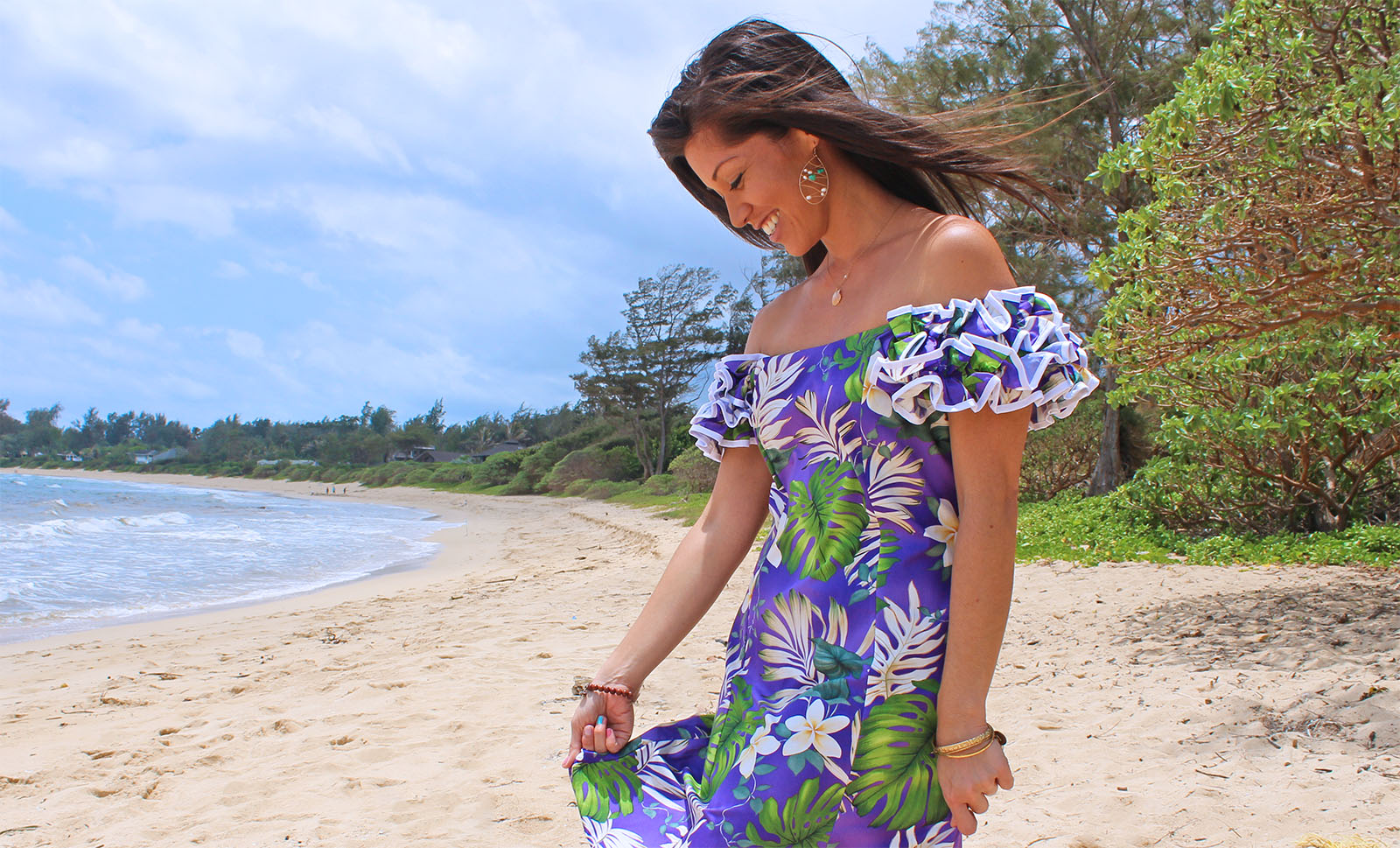In the foreground, a young woman stands as the focal point of the image, centered on a white sandy beach with the tide beginning to roll in on the left side. The woman appears tall and slender with medium brown skin and long, dark brown hair that lightens to a caramel hue at the ends. Her hair flows gracefully as she smiles, her eyes closed and head slightly tilted downwards.

She is adorned with teardrop-shaped earrings made of gold wire, interspersed with turquoise and pearl beads, and a matching turquoise and gold bracelet. Her gold necklace features a delicate pearl and a small golden clam. Her fingernails are painted turquoise to match her earrings.

The woman wears a dark purple dress with a gradient to light purple, decorated with patterns reminiscent of Hawaiian flowers and green-and-white Montserrat leaves. The dress has puffy sleeves accentuated with white detailing, and it sits off her shoulders, gracefully framing her neckline. Her left hand rests by her side while her right arm extends outward, gently holding a part of her dress.

In the background, behind her, lush greenery and trees can be seen, evoking the sense of springtime renewal. There are also some discernible homes, blending into the natural landscape. The entire scene is in sharp focus, capturing the serene moment of the woman standing on the beach in clear, vivid detail.